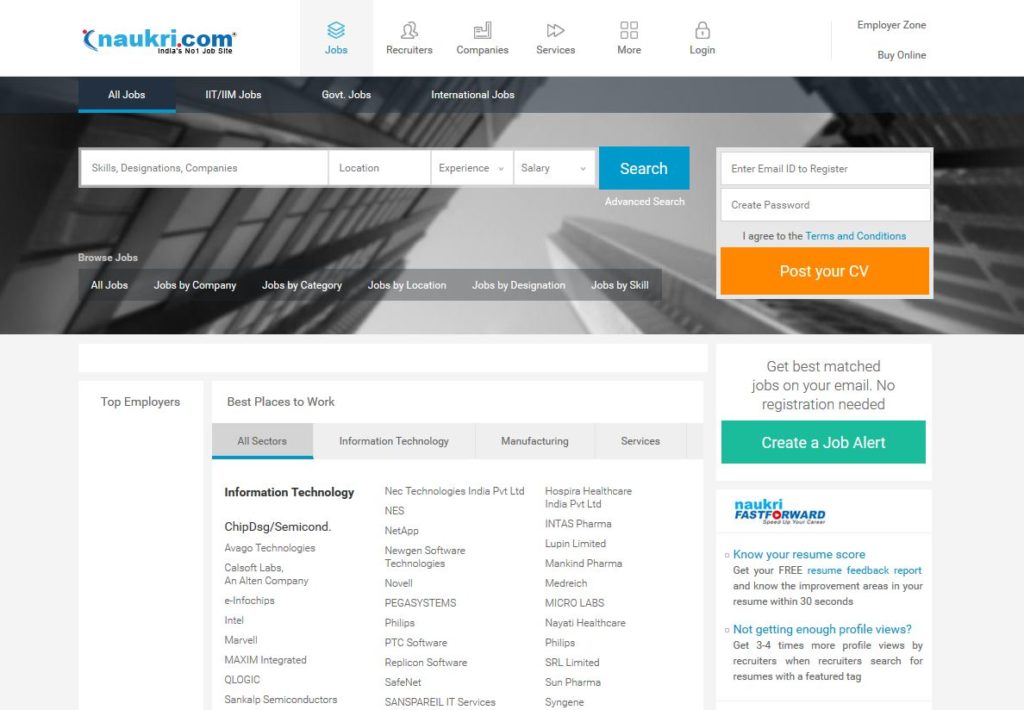This screenshot captures a webpage from Naukri.com, predominantly featuring a clean, minimalist design with a white and light-gray background. At the top left corner, the website logo appears in blue text reading “Naukri.com,” with the “com” portion in a darker blue hue. To the right of the logo, a navigation bar in gray text lists tabs: the first tab, “Jobs,” is highlighted in blue, followed by “Recruiters” paired with an icon of two people, then “Companies,” “Services,” “More,” and “Login.”

Below the navigation bar, a prominent rectangular image spans the width of the page, displaying a cityscape against a sky, with visible buildings on both the left and right sides. Within this image, at the top left, lies a long white rectangular search box featuring several input fields: "Skills, Designations, Companies" on the far left, then "Location," "Experience," and "Salary" sequentially. To the right of these fields is a prominent blue search button with white text reading “Search.”

At the bottom of the page, a series of white boxes with black text provide various pieces of information. Centrally located is a box titled “Best Places to Work,” under which there are four tabs labeled “For All Sectors,” “Information Technology,” “Manufacturing,” and “Services,” with the “For All Sectors” tab currently selected. Below this section, additional lines of black text enumerate different types of technology.